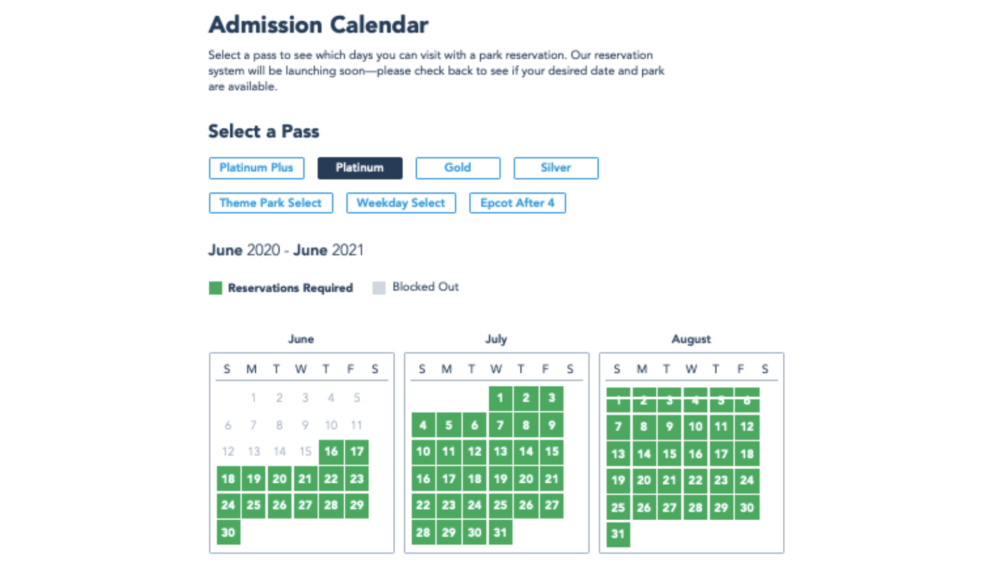Here is a cleaned-up and detailed caption for the image described:

---

The image is an interface of an application designed for purchasing amusement park passes or tickets. The top header reads "Admission Calendar," followed by the instruction, "Select a pass to see which days you can visit. Our reservation system will be launching soon. Please check back to see if your desired date and park are available."

Below this, there is a section titled "Select a Pass," featuring several pass options: Platinum Plus, Platinum, Gold, Silver, Theme Park Select, Weekday Special, and Epcot After 4. Each option is outlined in blue rectangles with the names listed in blue text inside the outlines. Currently, the "Platinum" pass is selected.

The date range displayed spans from June 2020 to June 2021. The interface includes three mini-calendar thumbnails for the months of June, July, and August. Each day on these calendars is color-coded: green signifies "Reservation Acquired," and white indicates "Blocked Out."

For June, dates from the 1st to the 15th are marked white (blocked out), while dates from the 16th to the 30th are green (available). For July, the entire month is available (all dates are green). Similarly, August is entirely available, though dates from the 1st to the 6th feature a line through them yet remain green, indicating a special condition that is not explicitly clarified within the interface.